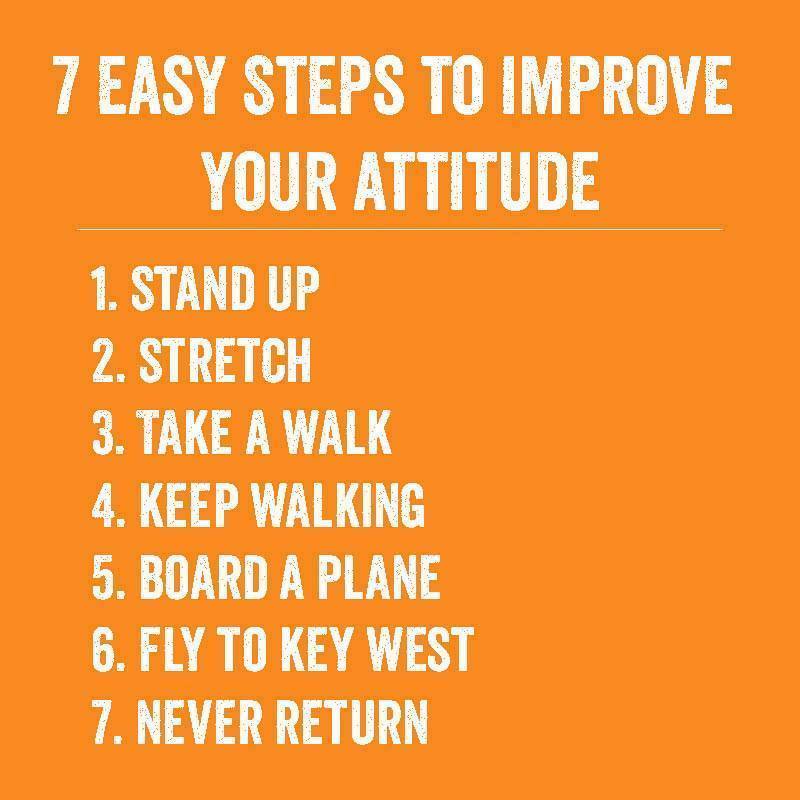The image is a square graphic resembling an Instagram post, featuring a vibrant orange background with prominent white, bold, all-caps text in the center. At the top, it reads, "SEVEN EASY STEPS TO IMPROVE YOUR ATTITUDE," with a thin horizontal white line underscoring the title. Below this line is a numbered list of seven steps, each in large, white bold letters. The steps are: 1. Stand up, 2. Stretch, 3. Take a walk, 4. Keep walking, 5. Board a plane, 6. Fly to Key West, and 7. Never return. The playful steps suggest a whimsical approach to boosting one's mood through an impromptu escape, perhaps hinting at an advertisement for travel to Key West.